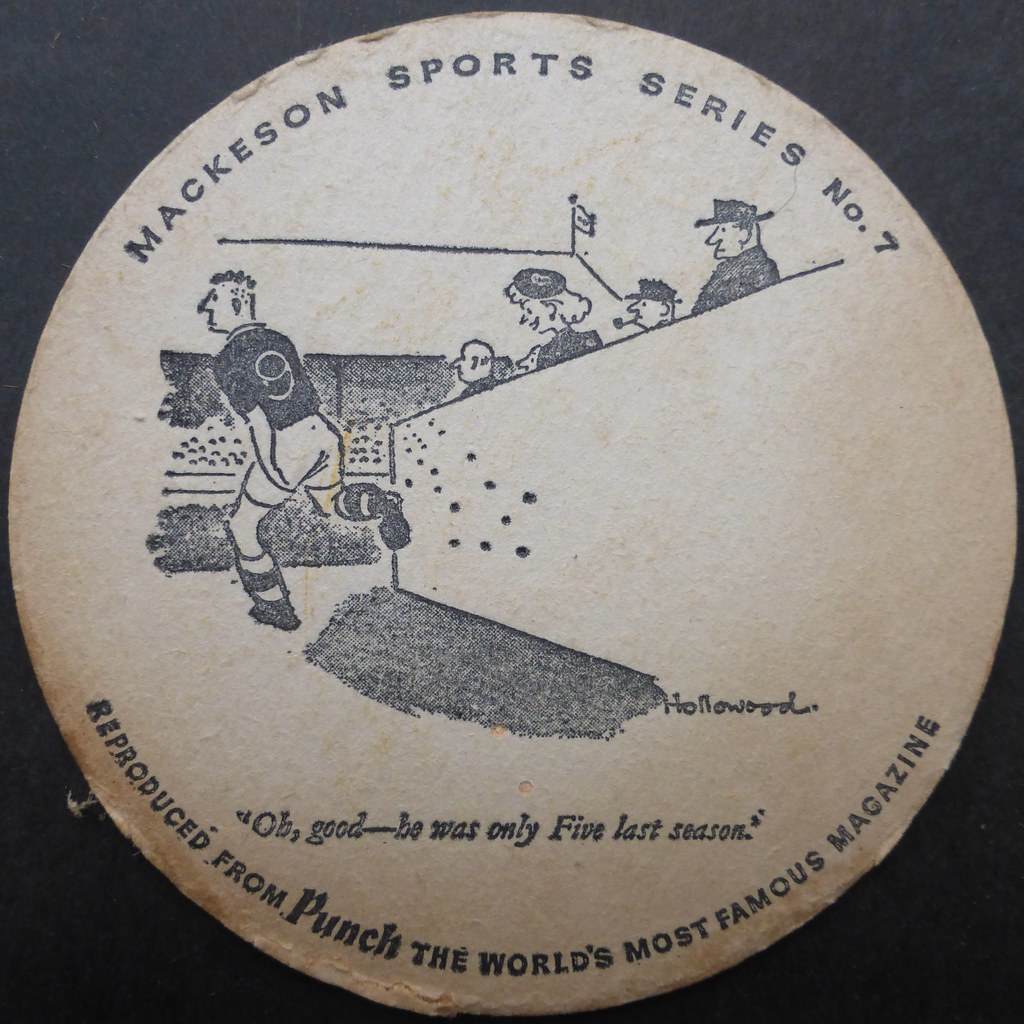This image features a vintage, black-and-white illustration combined with typography, all centered on a black square background. It resembles an old pin or a magazine clipping. The main element is a faded, white circle with black lettering curving around its top edge, reading "Mackeson Sports Series No. 7". Within the circle is a detailed sketch from what appears to be the 1940s or 1950s, depicting a soccer player wearing a number nine shirt, white shorts, and striped leggings, running onto a soccer field. To his right, several spectators, including a gentleman in a hat with a pipe and a smiling woman in a pillbox hat, are watching from the stands, which are dotted with more viewers in the background. Below this scene, in italicized quotations, is the humorous caption, "Oh good, he was only five last season." At the bottom of the circle, the text "Reproduced from Punch, the world's most famous magazine" is inscribed, attributing the illustration to the renowned publication. The overall style is reminiscent of vintage collateral print, reflecting a nostalgic sports moment.